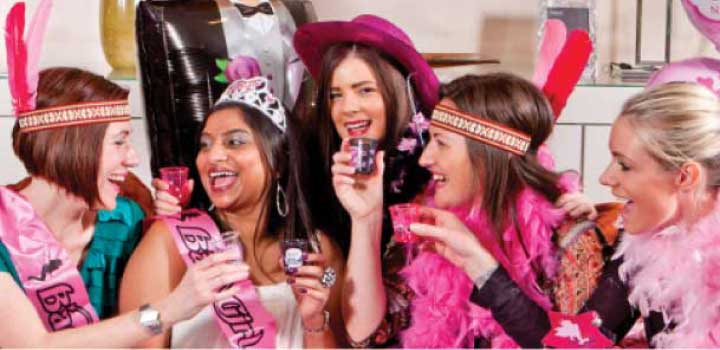This vibrant image captures a joyous indoor bridal party featuring five young women, gathered around and celebrating with the bride at its center. The bride, who appears to be of ethnic descent with darker skin and features, stands out with a silver and pink bridal crown on her head, an extravagant cocktail ring on her finger, and a white shirt with a pink ribbon draped across her chest. She holds a shot glass in her left hand, her expression animated and joyful as she laughs and engages with a friend to her right who is cheering her with another shot glass. This friend, a white woman with short red hair, is adorned with a playful headband featuring pink feathers and a vibrant green top with a pink ribbon.

To the bride’s left, there is another woman with a cowboy hat on, bright pink in color. She is dressed in black and stands in front of a whimsical balloon decoration shaped like a person in a tuxedo. Continuing the line, a woman with short brown hair wears a headband with pink and red feathers; she sports a shot glass and a playful arrangement of lulas around her neck. On the far right, another blonde woman holds a pink shot glass, complemented with a lighter pink lula around her neck. The group, composed of four white women and the bride, who is likely Latina, are all smiling and cherishing the moment together within a room dominated by white walls, bright outfits, and cheerful decor, signaling a lively and festive occasion.